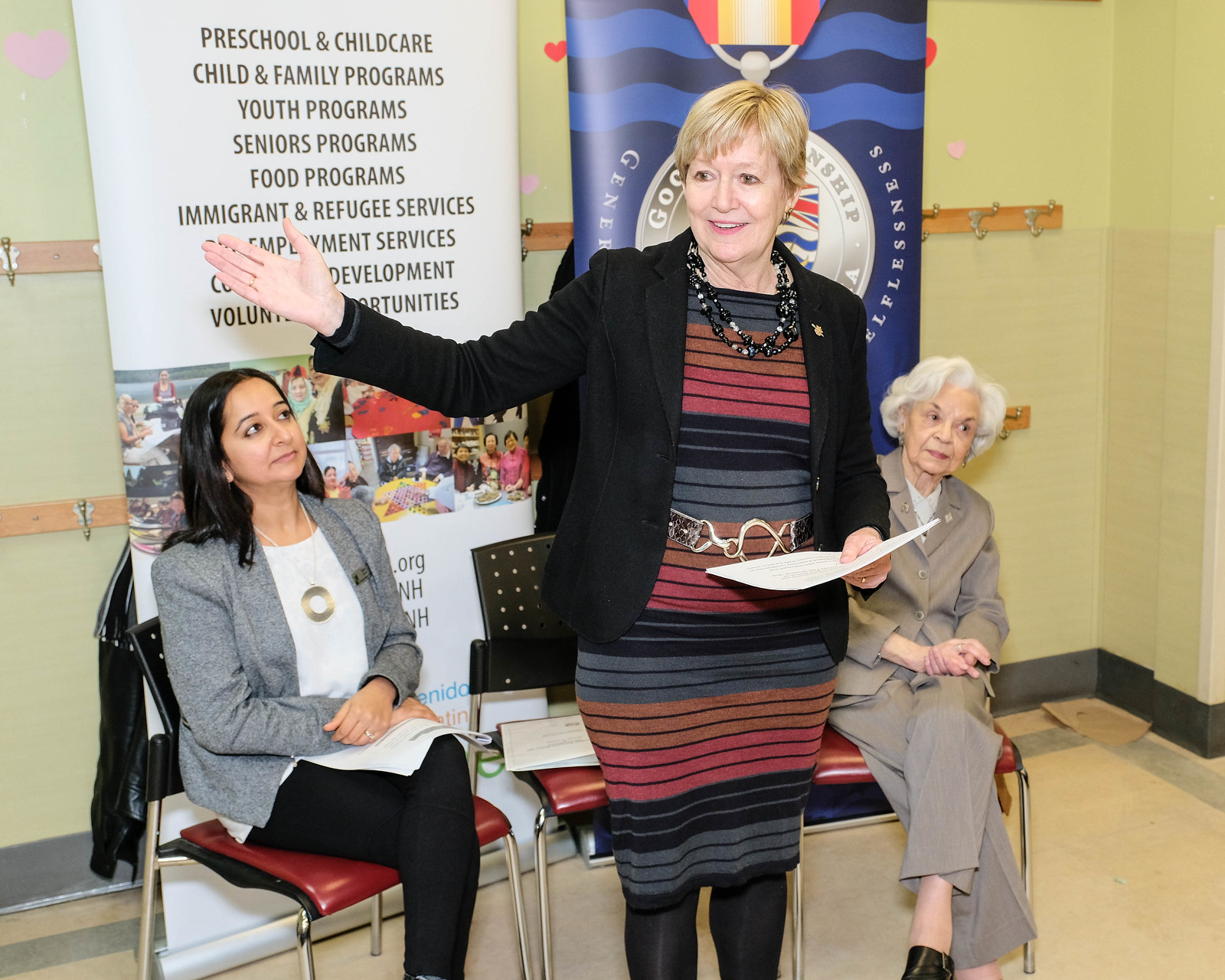This photograph captures a moment during a presentation involving three women, each distinctly described. At the center, a blonde woman in her 40s, with short hair cascading to her ears, stands addressing the room. She dons a black jacket adorned with a pin and wears two beaded necklaces over a vibrantly-striped dress in shades of gray, black, pink, and orange. Her outfit is completed with black stockings and she holds a piece of paper, suggesting she's speaking or leading the presentation.

Seated beside her, two women are positioned in black metal chairs with red cushions. To the right, an elderly woman with white hair is elegantly dressed in a tan-colored suit, sitting cross-legged. On the left, a brunette looks upward at the standing woman, her attire consisting of a gray jacket over a white blouse paired with black pants.

The backdrop features two banners. One highlights services and programs such as Preschool and Child Care, Child and Family Programs, Youth Programs, Senior Programs, Food Programs, and Immigrant and Refugee Services. The second, though harder to discern, is prominently blue and displays what appears to be a large medal or award hanging from it.